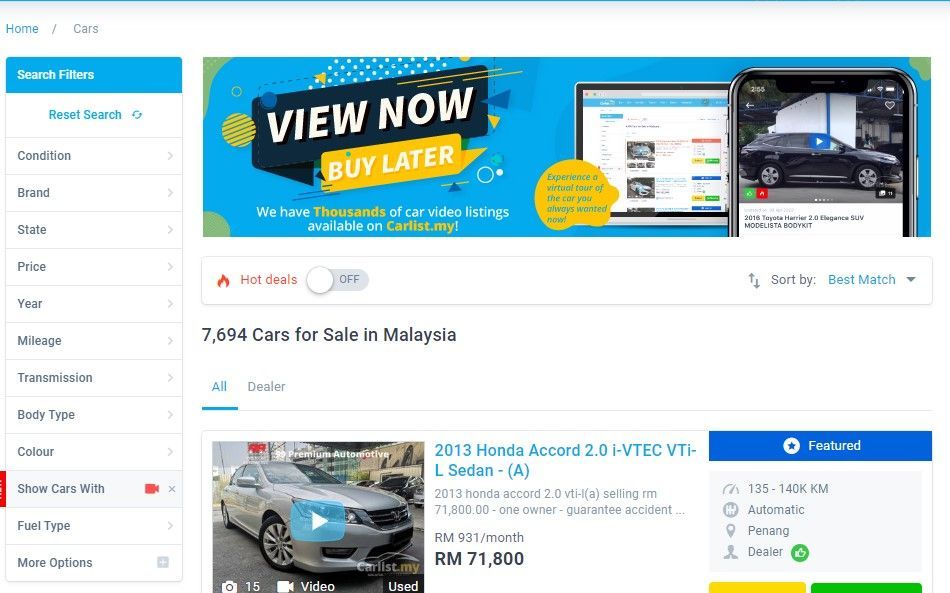Screenshot of an online car marketplace:

At the top of the screen, the breadcrumb navigation reads "Home / Cars." A prominent blue button labeled "View Now, Buy Later" encourages users to explore the thousands of car video listings available on Carless.my. The banner reads, "Experience a virtual tour of the car you've always wanted now."

Below this header, there is a section for sorting options, with "Hot Deals" turned off and "Sort by Best Matches" selected. A tally indicates there are 7,694 cars for sale in Malaysia. Filtering options include "All" or "Dealer," with "All" currently selected (underlined).

The featured car listing showcases a 2013 Honda Accord 2.0 i-VTEC VTIL sedan. The listing specifies details such as:

- Model: 2013 Honda Accord 2.0
- Price: RM 71,800
- Financing: RM 931 per month
- Ownership: One owner, guaranteed accident-free
- Mileage: 135,000 - 140,000 km
- Transmission: Automatic
- Dealer: Endorsed with a thumbs up icon

There is also a "Featured" tag highlighted in blue with a star icon.

A yellow and a blue bar are displayed towards the bottom of the listing, likely indicating additional information or metrics.